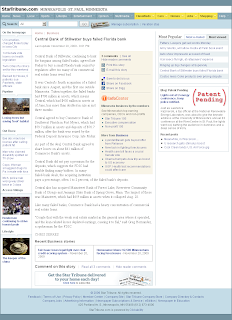The image is a small, indistinct screenshot of a website. Due to its limited size, the text is unreadable. At the top of the webpage, a search bar is faintly visible, suggesting the ability to browse different categories. Below the search bar, there appears to be an article section filled with text, interspersed with images to the left. In the center-right area of the page, there is a noticeable pale yellow box, possibly highlighting important information or serving as an advertisement.